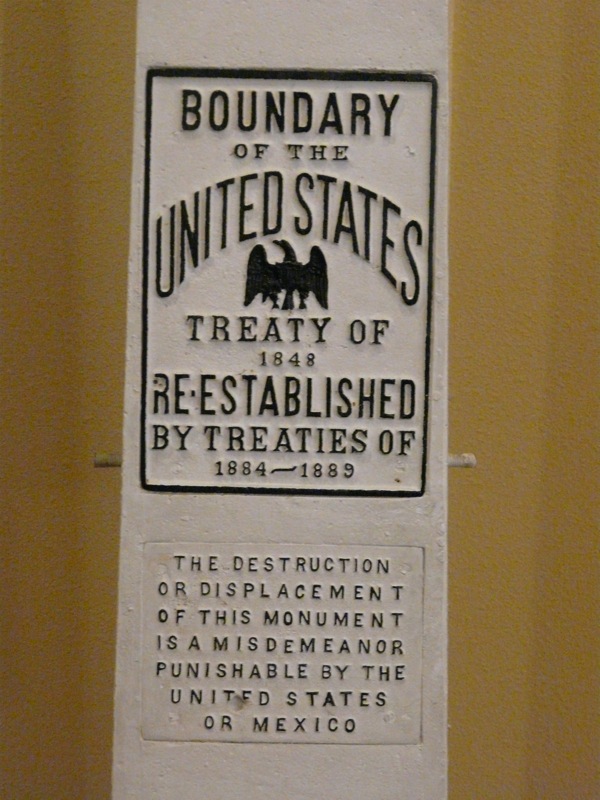The image depicts a close-up of a boundary marker for the United States, set against a yellowish painted wall. The marker is a tall, narrow, white vertical rectangle with a black rectangular section towards the top. The black section has the inscription "Boundary of the United States" in black lettering. Below the inscription is a black silhouette of an eagle with its wings spread and head facing to the left. Underneath the eagle, the text reads "Treaty of 1848, reestablished by treaties of 1884-1889." Beneath this, another area with a thin black border contains the warning: "The destruction or displacement of this monument is a misdemeanor punishable by the United States or Mexico." The white background and black text create stark contrast, making the text easily legible. The overall shape and design of the marker resemble a utility pole, suggesting it may have elements that extend outwards, akin to climbing rungs used by electricians or construction workers.